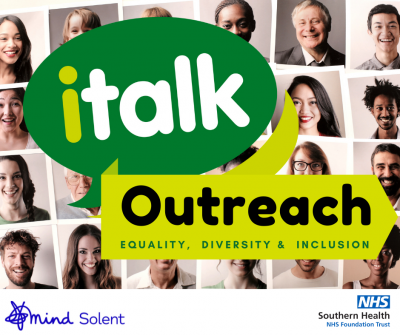In the image, the top-left corner features a prominent, large green speech bubble containing the text "I talk” in light green, with "talk" in white. Positioned to the bottom right of this is another speech bubble; it is rectangular with a pointed arrow on the right side, colored light green, and inside it reads "outreach" in black.

Beneath these, in dark green text, are the words "equality, diversity, and inclusion." The background showcases four rows of profile pictures, each row containing approximately six images, featuring people of varied ethnicities, ages, and genders, embodying a diverse and inclusive community.

In the bottom right corner, there is a blue rectangle with white text that reads "NHS," and below it, "Southern Health NHS Foundation Trust." In the bottom left corner, there is a logo resembling a star that extends rightward into the cursive word "Mind," followed by the word "Solid," all in dark blue. The majority of the background is white, connecting between the portrait pictures and behind the logos of NHS and Mind Solid. Overall, this image integrates messages of communication, outreach, and inclusivity with visual diversity prominently displayed.